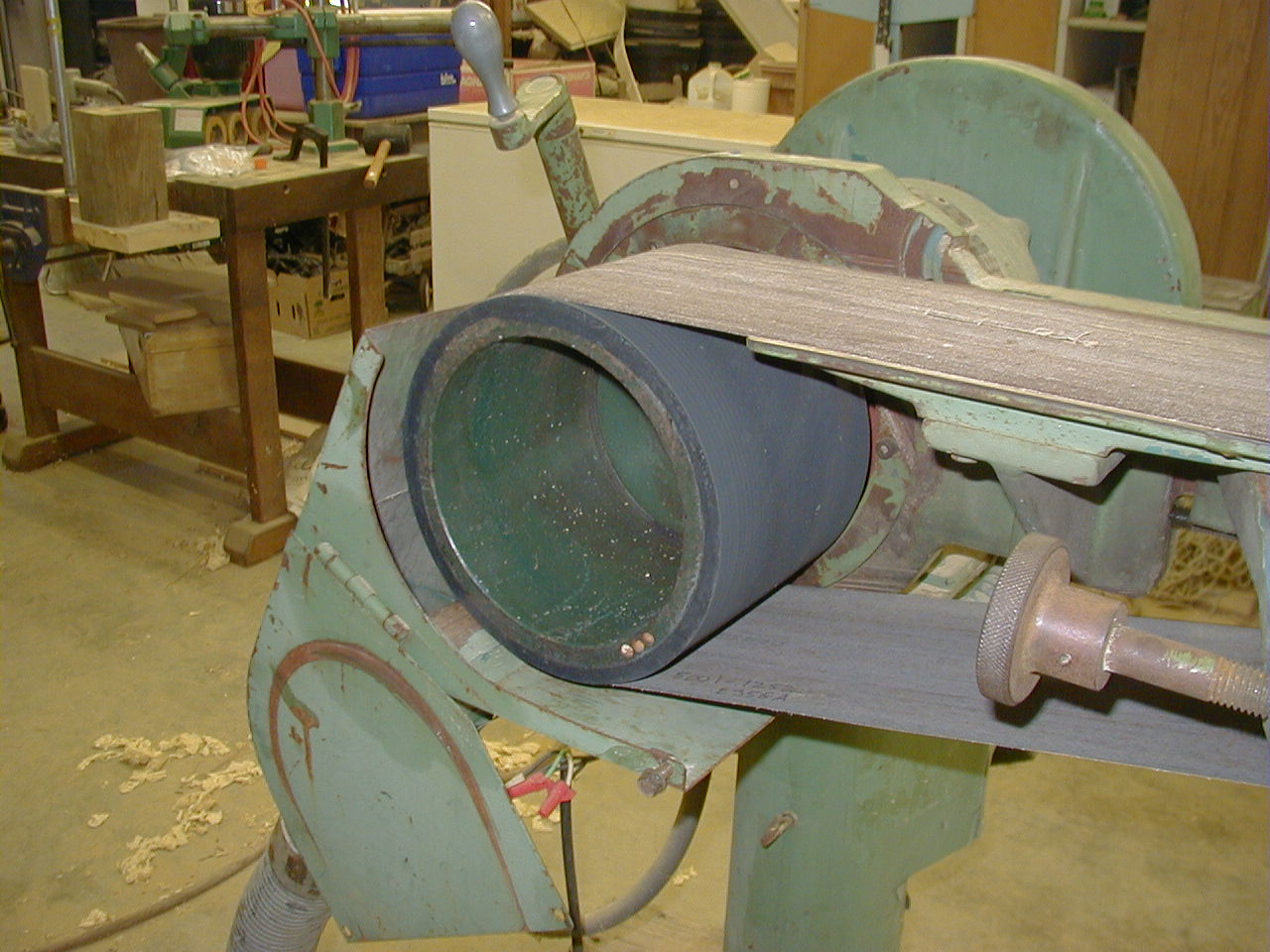The photograph captures a well-used industrial sanding machine prominently set in a workshop. The large green piece of machinery features a significant amount of worn and chipped paint, revealing rust beneath, indicating its age and extensive use. Dominating the machine is a large black cylinder enveloped by a grainy-textured sanding belt that extends off-screen. To the rear of the machine, a robust rod is fitted with a gray, bulbous-shaped knob. The workshop setting is further emphasized by an unfinished concrete floor scattered with white debris, possibly paper or cloth. Background elements include scattered cardboard and wooden boxes, wooden workbench cluttered with additional tools and materials, a rubber mallet, wood blocks, as well as various shelves and equipment running across the frame from left to right. Despite the evident clutter and wear, the area exudes a sense of practical functionality.